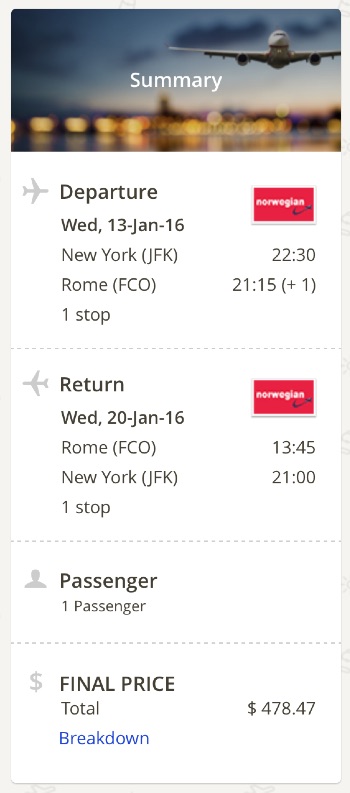This image is a detailed screenshot of a flight itinerary summary. At the top, the word "Summary" is prominently displayed in white text against a backdrop featuring an aircraft either descending or ascending closely above the runway at night, with runway lights illuminated to guide the pilot.

Beneath this banner are the details of the itinerary. The departure flight is scheduled for Wednesday, January 13th, 2016, leaving from New York at 22:30 (10:30 PM) and arriving in Rome at 21:15 (9:15 PM), with just one stop en route. The return flight is set for Wednesday, January 20th, 2016, departing from Rome at 13:45 (1:45 PM) and landing back in New York at 21:00 (9:00 PM). The itinerary is for a single passenger, with a total cost of $478.